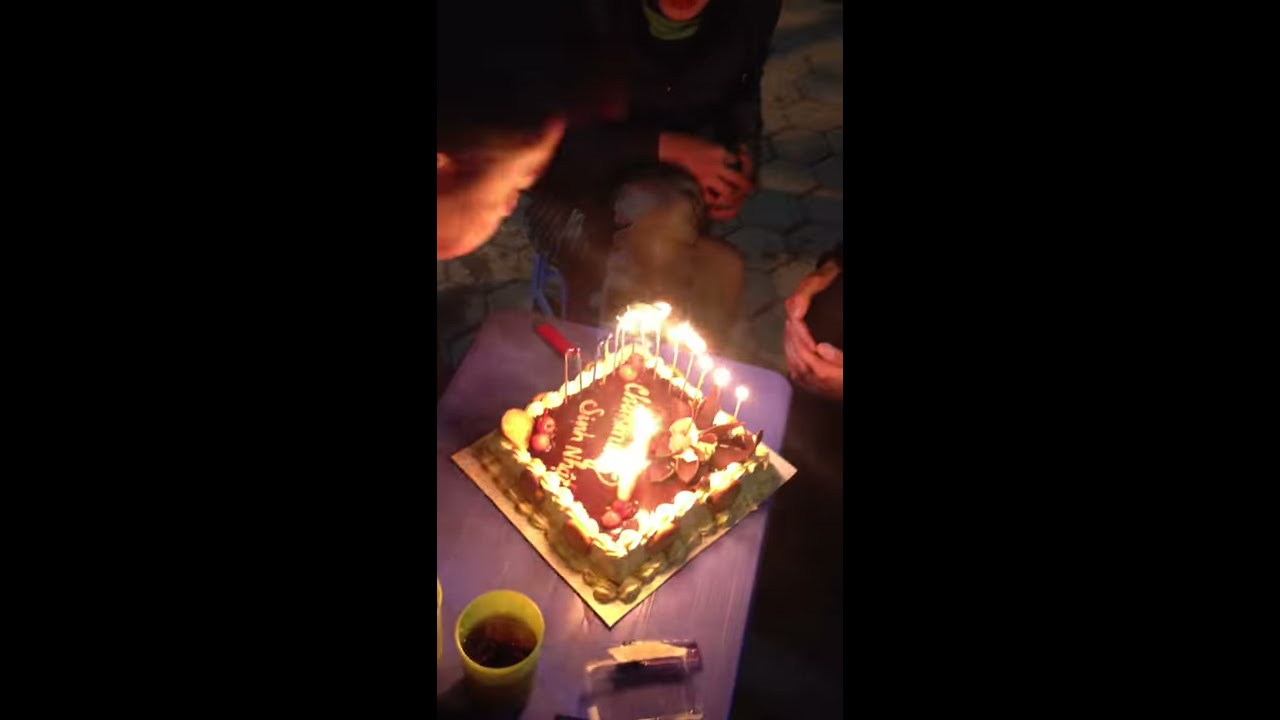In this indoor image, a birthday celebration is captured with a detailed focus on a central cake. The cake is a square, chocolate-brown delight with white scalloped frosting along its edges and lit candles adorning its corners. One of the main decorations is a chocolate flower positioned on a corner, accompanied by strawberries on the remaining three corners. The top of the cake features white frosting text, all sitting atop a flat piece of cardboard on a low rectangular purple table. A green cup, partially filled with a dark liquid that resembles Coke, is placed nearby. To the left of the cake, a red lighter rests on the table. The scene is dimly lit, highlighting the flickering candles and the face of a person in the upper left corner, who is in the process of blowing out the candles. Additional people surround the table, though only parts of their bodies and hands are visible in this celebratory moment.